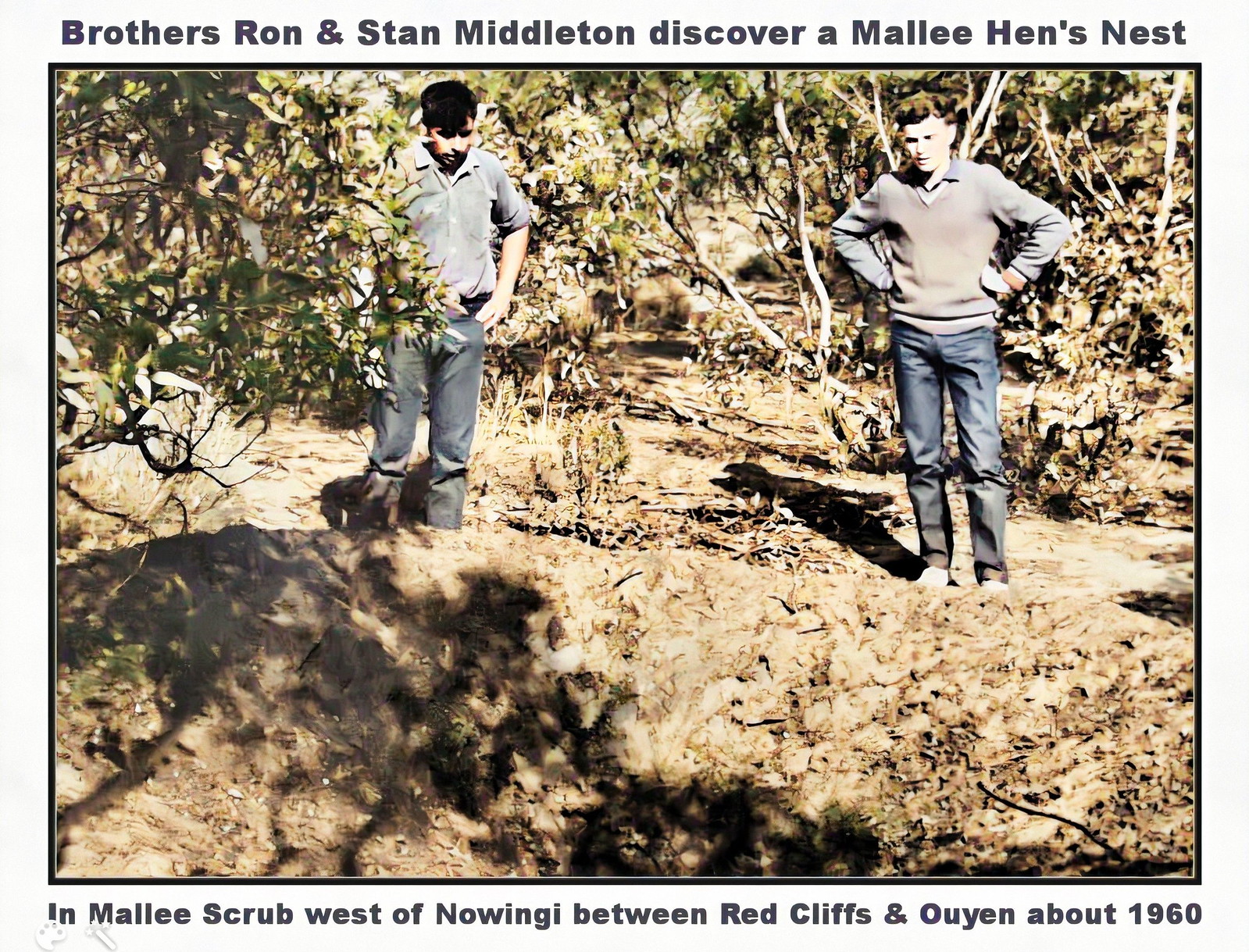In this 1960 photo, brothers Ron and Stan Middleton are captured in a moment of discovery as they examine a mallee hen's nest in the mallee scrub west of Nowing Eye, between Red Cliffs and Oyen. The image, bathed in bright sunlight, portrays an arid Australian landscape with dirt, leaves, and numerous trees. Both men are casually dressed in blue jeans; Ron, on the left, sports a gray polo shirt with rolled-up sleeves, while Stan, on the right, wears a gray long-sleeve shirt and holds his hands on his hips. They stand over what appears to be a large ditch, intently looking down, although the nest itself is not visible. A shadow of a tree stretches across the scene, and the image is framed with a light, almost white border. Text on the top and bottom borders identifies the event and location, adding historical context to this evocative snapshot of rural life in the Australian outback.